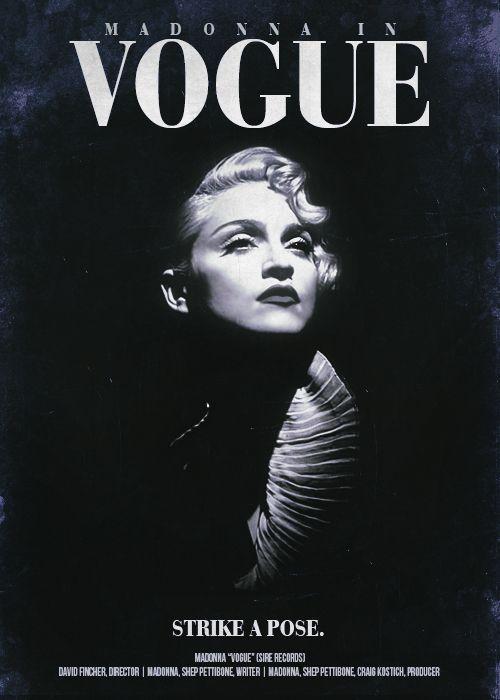The image appears to be a vertically aligned rectangular poster with a primarily black background, subtly faded to gray in the upper left and right corners. Centered at the top, the poster prominently displays the text "MADONNA IN" in all caps, written in beige serif font. Below, the word "VOGUE" is featured in large, block beige letters. This text is followed by a black-and-white image of a younger Madonna with asymmetrical short hair, styled with one side combed over and curled down, and wearing dark lipstick. Beneath her image, the phrase "STRIKE A POSE." is displayed in bold, all caps white text.

Further down, centered at the bottom in smaller caps, it reads "MADONNA VOGUE" in quotes, followed by "(SIRE RECORDS)." Listed below this are the credits, separated by vertical lines: "DAVID FINCHER, DIRECTOR | MADONNA, SHEP PETTIBONE, WRITER | MADONNA, SHEP PETTIBONE, CRAIG KOSTICH, PRODUCER." The entire poster emits a sophisticated yet edgy aesthetic, reflective of Madonna's iconic style and the timeless appeal of her hit song "Vogue."